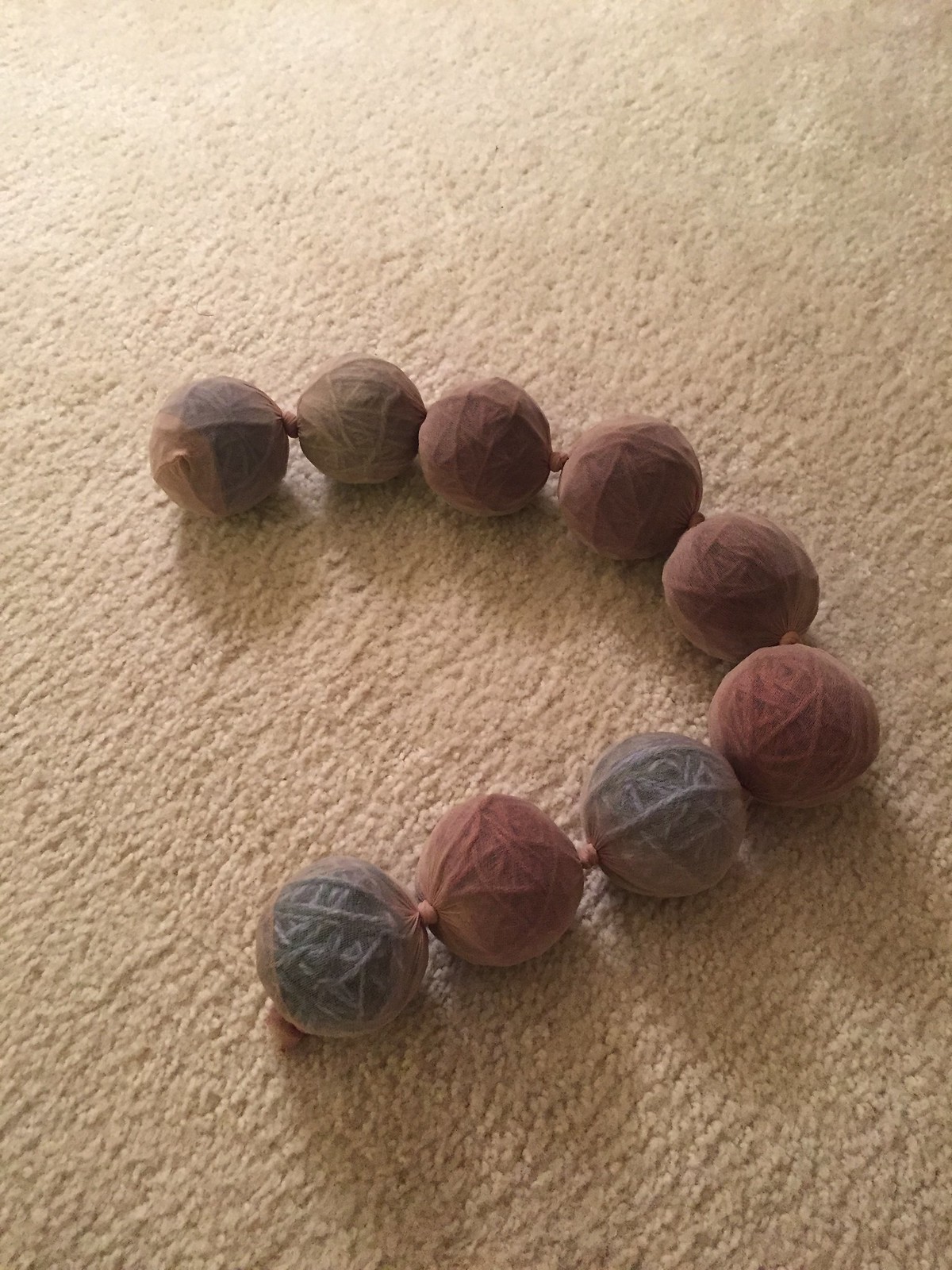This detailed color photograph captures a series of nine interconnected balls lying on a well-worn beige carpet. The carpet appears to be either textured from extended use or composed of a short-pile material. The balls are arranged in a curved line resembling a lowercase 'n', casting faint shadows on the carpet beneath them. These intriguing spheres seem to be wrapped in thin layers of material, either resembling yarn or translucent pantyhose, giving them a distinctive look akin to beads on a string or a disconnected rosary. The spheres boast a varied palette, including shades of gray, dark dusty rose, brownish hues, olive, and combinations of purple, red, orange, and white, although the exact colors appear somewhat muddled due to the lighting. The meticulous arrangement and the unusual material suggest a homemade or artistically crafted object.